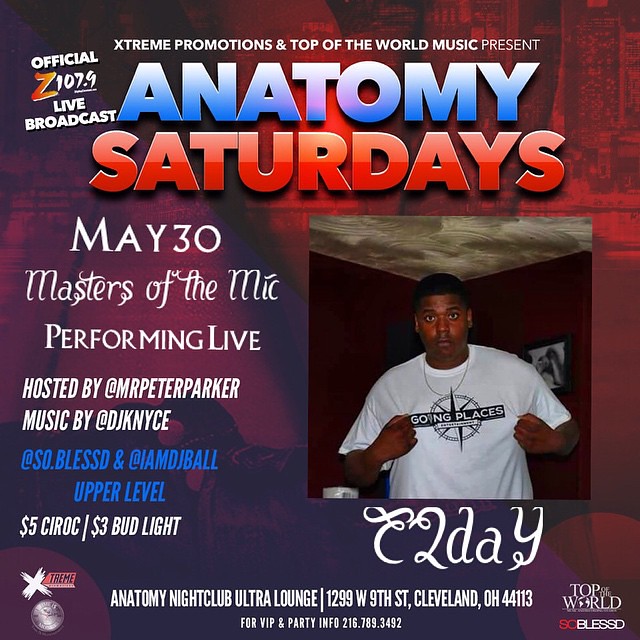The flyer, designed to promote a nightclub event, features a headline reading "Anatomy Saturdays" with "Anatomy" in a blue gradient and "Saturdays" in a red gradient. Above this, in small white letters, it states "Extreme Promotions and Top of the World Music present." At an angle in the top left corner, a logo declares "Official Z107.9 Live Broadcast." An image on the right side depicts an African American man in his 30s, facing the camera and holding his white t-shirt, which features a black nautical star and the words "Going Places." Below this, it reads "Easy Day." 

The center-left portion of the flyer details the event happening on May 30th, named "Masters of the Mic Performance Live," hosted by Mr. Peter Parker with music by DJ Nice (NYCE). It also mentions performances by "So Blessed" and "I Am DJ Ball" on the upper level. Promotional drink prices are highlighted with "$5 Ciroc" and "$3 Bud Lights." 

At the bottom, the flyer provides further information about the Anatomy Nightclub Ultra Lounge, including its address in Cleveland, along with several logos. The background gives off an industrial, gritty vibe, complementing the photographic and graphic design elements of the flyer.